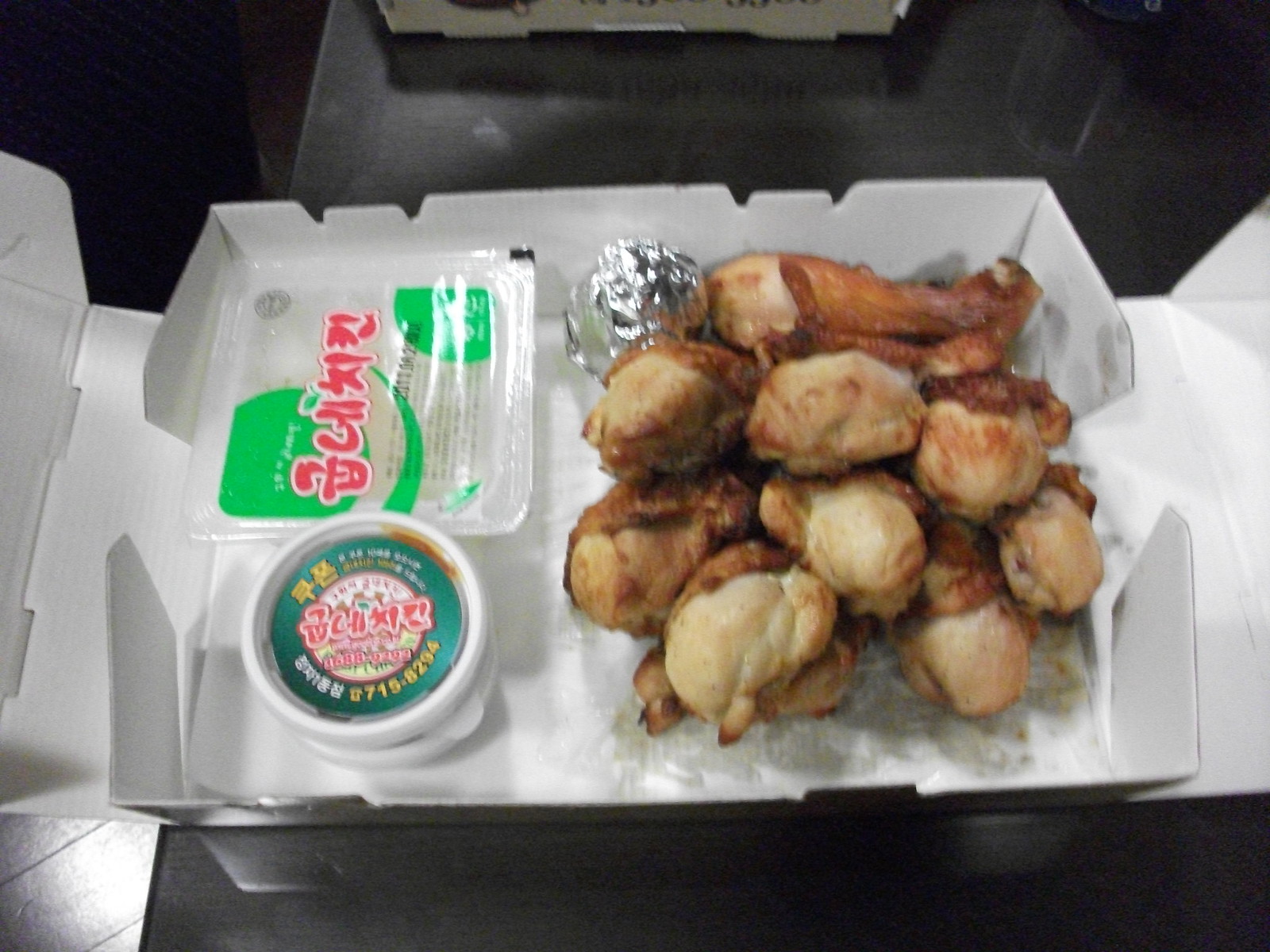This photograph depicts a slightly blurry image of food in a white, flat cardboard takeout container resting on a black surface. The primary focus on the right-hand side of the container appears to be several pieces of fried chicken wings or similar meat, characterized by their brown coloration and associated grease stains visible at the bottom. At the top edge of the container, near the meat, is a small ball of aluminum foil. To the left of the meat is a square packaged food item with a clear and green plastic peel-off lid, featuring Asian lettering in red and black, possibly indicating a brand name. Below this is a circular condiment cup with a lid adorned in green, yellow, and red designs, showcasing the same red characters. The container may be situated on a restaurant counter, inferred from the visible white tile flooring in the background.